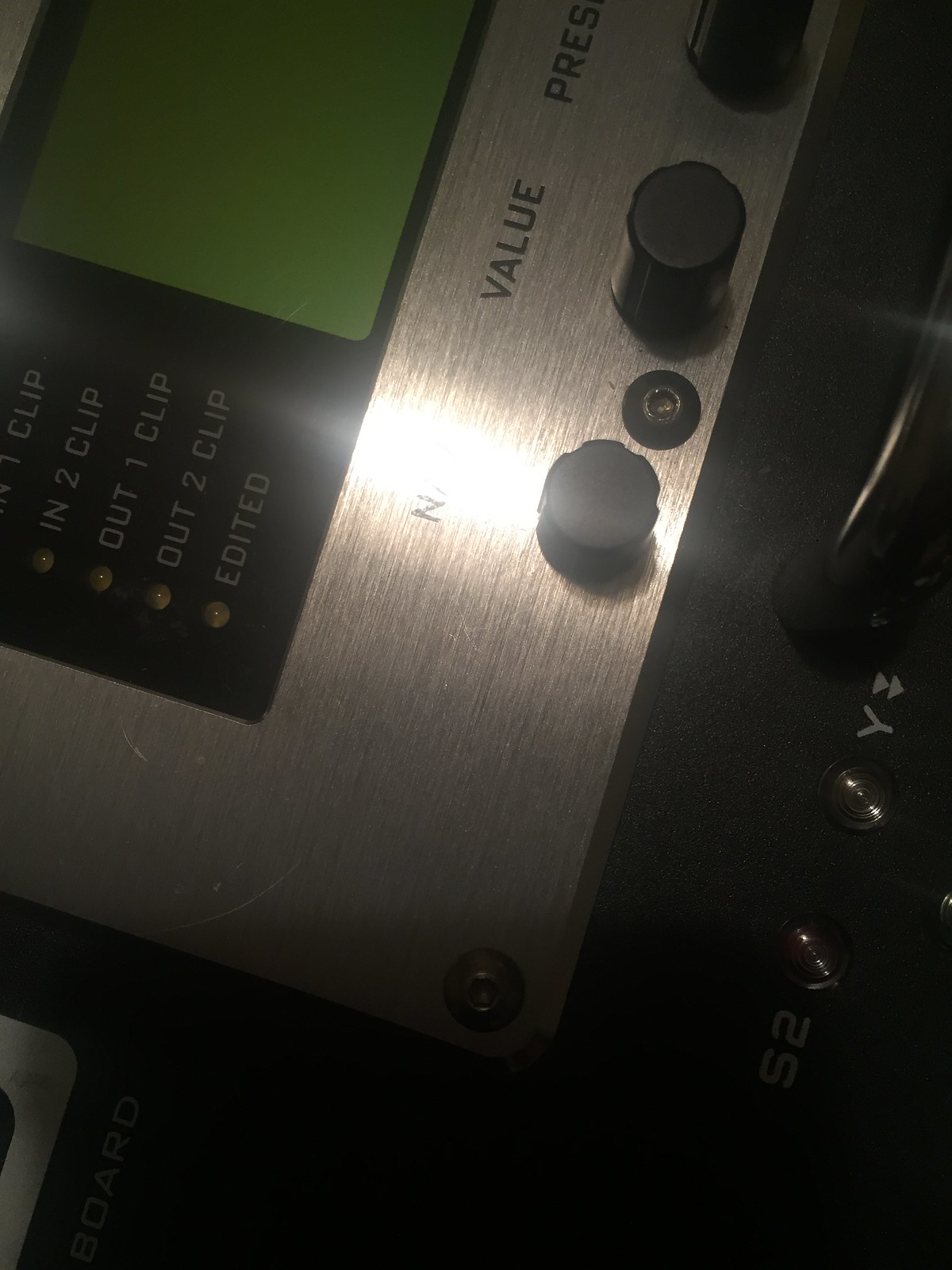The photograph features a poorly lit piece of equipment that appears to be some sort of audio or video control board. The silver control panel, which extends mainly vertically before making a left turn, is adorned with three knobs. The first knob, partially obscured by glare, is labeled with the single letter "N." The subsequent knobs are clearly marked "value" and "preset." Adjacent to these, a green LCD screen, currently unlit, is surrounded by five LED indicators. These LED indicators are labeled as "in one clip," "in two clip," "out one clip," "out two clip," and "edited." The photograph also highlights a black component near the screen and multiple black wires extending from the bottom of the device. The entire unit is riveted together, and a small text reads "board" on the panel. The image suggests a functional piece of equipment, possibly for professional audio or video recording.